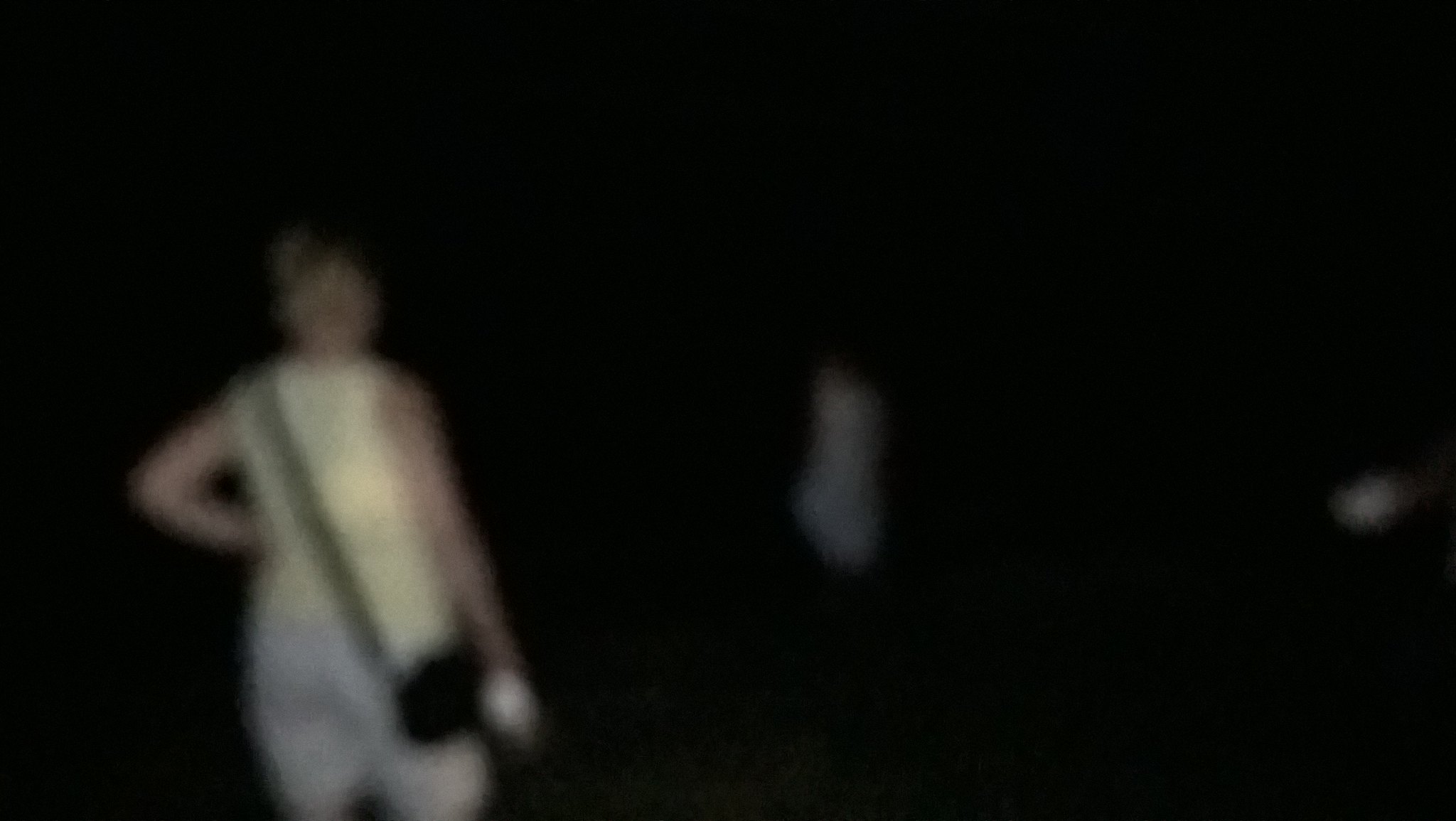This is a highly dark and blurry image that depicts two individuals standing outdoors, presumably in a grassy area, possibly a lawn or a wilderness setting, under minimal lighting conditions. The photograph appears to have been taken in almost pitch-black darkness, suggesting that the camera used did not have an adequate flash, resulting in an unclear light source that illuminates the subjects.

At the top of the image, there is nearly complete darkness. Moving downwards, the vague outlines of the people become slightly discernible. On the right side of the image, there's an indistinct, whitish blur, its nature remaining unidentified.

In the foreground stands a woman with short blonde or brown hair. She is wearing what appears to be a white sleeveless shirt and possibly blue pants. Over her shoulder, she has a fanny pack, characterized by a black strap. Her right hand is confidently placed on her hip.

In the background, the shadowy figure of another person can be seen, dressed in what looks like white or blue clothing, though the details remain indistinct due to the poor lighting conditions of the image.